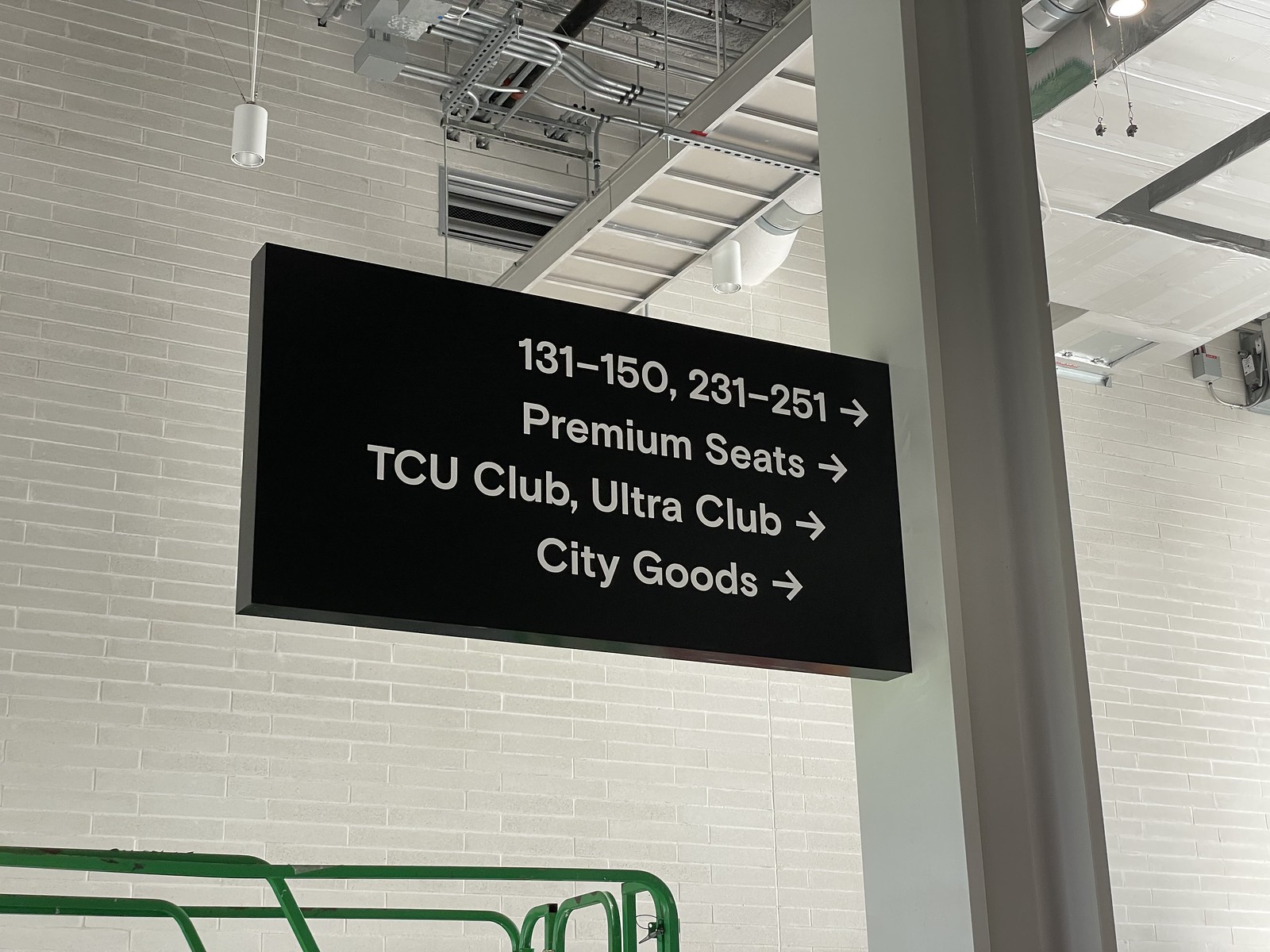The detailed image showcases a black sign with white text attached to a light green metal pole, positioned against a white brick wall backdrop. The sign consists of four lines of text, each ending with an arrow pointing to the right. The first line reads "131-150, 231-251." The second line states "Premium Seats." The third line mentions "TCU Club, Ultra Club," and the final line indicates "City Goods." Surrounding the sign is an industrial setting featuring a white canister light hanging from the ceiling, additional silver metal piping, hanging wires, and another light fixture. The setting appears to be inside a stadium, characterized by an absence of windows and a fully covered industrial roof. The green banister is noticeable on the lower left-hand side of the image.